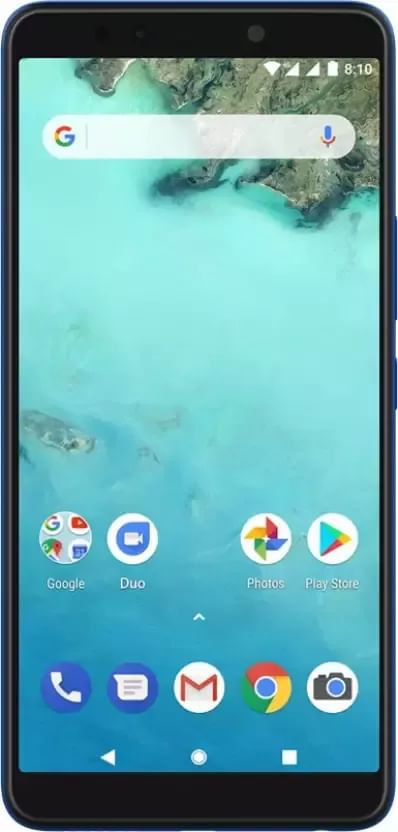The image features a Google phone, possibly in black or dark blue, though the exact color is uncertain. The screen displays the device's full battery and the current time, 8:10. The phone's wallpaper captures a picturesque scene of shimmering blue ocean water with a hint of volcanic rock, resembling a remote, uninhabited island akin to those found in Hawaii.

Dominating the top portion of the screen is the Google search bar, complete with the Google logo, a blank space, and a microphone icon. Below this bar, there is ample blank space leading down to the app icons. The first row features Google apps: Google, Duo, Google Photos, and the Play Store. At the very bottom of the screen, additional icons are visible for essential functions: phone calls, text messaging, Gmail, Google Chrome, and the camera.

The navigational buttons are displayed at the bottom: a white circular home button in the center, a white square representing the app drawer to its right, and a white back arrow to its left. This clear arrangement of Google-related apps and the overall design unmistakably identify the device as a Google phone, distinctively not an iPhone.